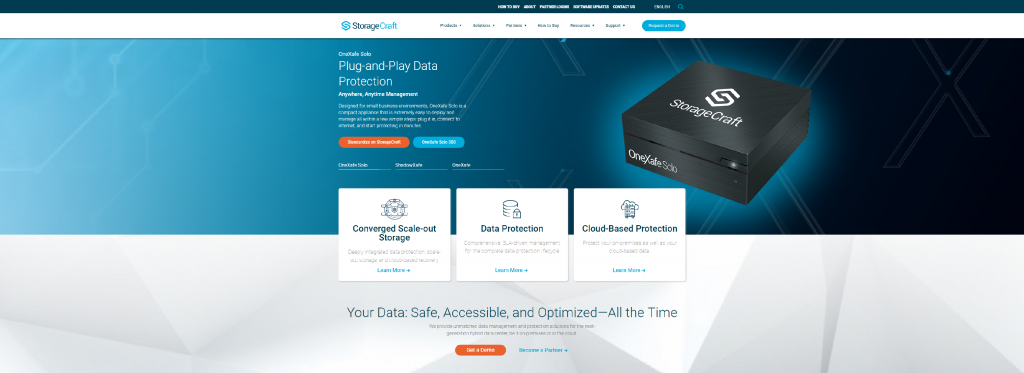The website belongs to a company called StorageCraft. At the top, there's a white navigation bar with small, readable categories that offer drop-down menus. Above this, a black bar spans the width of the page, featuring white text that is difficult to read due to its small size. Below the white bar, the phrase "Plug and Play Data Protection" is prominently displayed, though other text around it is similarly too small to be decipherable.

The central part of the page is dominated by a large, long orange block positioned next to a similarly-sized blue block. Beneath these, three distinct sections describe the company's key offerings: "Converged Data Protection," "Scale-Out Storage," and "Cloud-Based Protection." Each section is accompanied by an image, a brief explanation, and a "Learn More" link in blue at the bottom.

An image showcasing the StorageCraft logo follows, revealing that the initial misreading of "Storage Out" was incorrect. The logo appears in a black box with a 3D-style white insignia.

Further down, a white box with gray shading reassuringly states, "Your data is safe, accessible, and optimized all the time," accompanied by a small, unreadable statement underneath. An orange box and blue text complete the page's visually engaging layout.